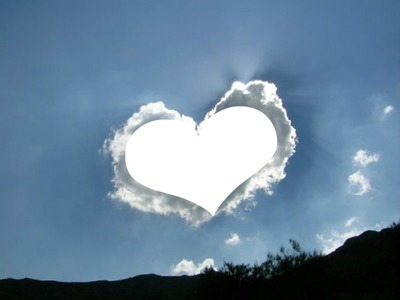The image captures a serene sky setting viewed from a ground perspective, and predominantly features a gradient blue sky with a light periwinkle hue. Dominating the image, from the top left to about 90% toward the bottom, is this expansive sky backdrop. A silhouette of dark trees or bushes spans across the bottom portion, creating a stark contrast with the bright sky above. Centered in the image, a white heart graphic overlays a heart-shaped cloud that is half gray and half white. Additional wispy clouds surround the heart, particularly to the bottom center and far right. Light emanates from this central cloud, brightening the surrounding sky, implying it's near the sun. The authenticity of the photograph is evident, barring the clearly artificial white heart graphic superimposed onto the natural cloud formation.